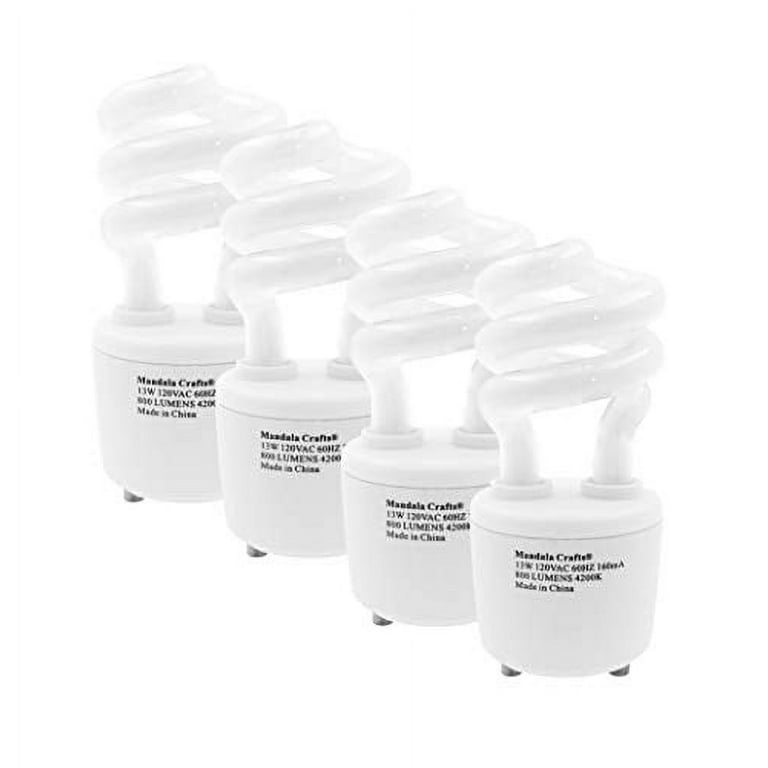This image features a set of four compact fluorescent lamps (CFL)—also referred to as LED bulbs by one of the descriptions—arranged diagonally from the center to the upper left against a white background. Each bulb is upside down, showcasing elongated, curved tubes that form a spiral pattern above their cylindrical white bases. These bases, approximately three to four inches in height, are detailed with black text that includes the partially readable "Mad Lala Crafts" or "Mandela Crafted," "12 watts," "120 volts," and "Made in China." Additionally, the bases have two silver contacts at the bottom. The intricate design of the tubes, described as resembling neon swirls, adds a distinct visual element to the bulbs, highlighting a blend of clear and white coloration in the glass parts that are designed to illuminate in a spiral pattern.